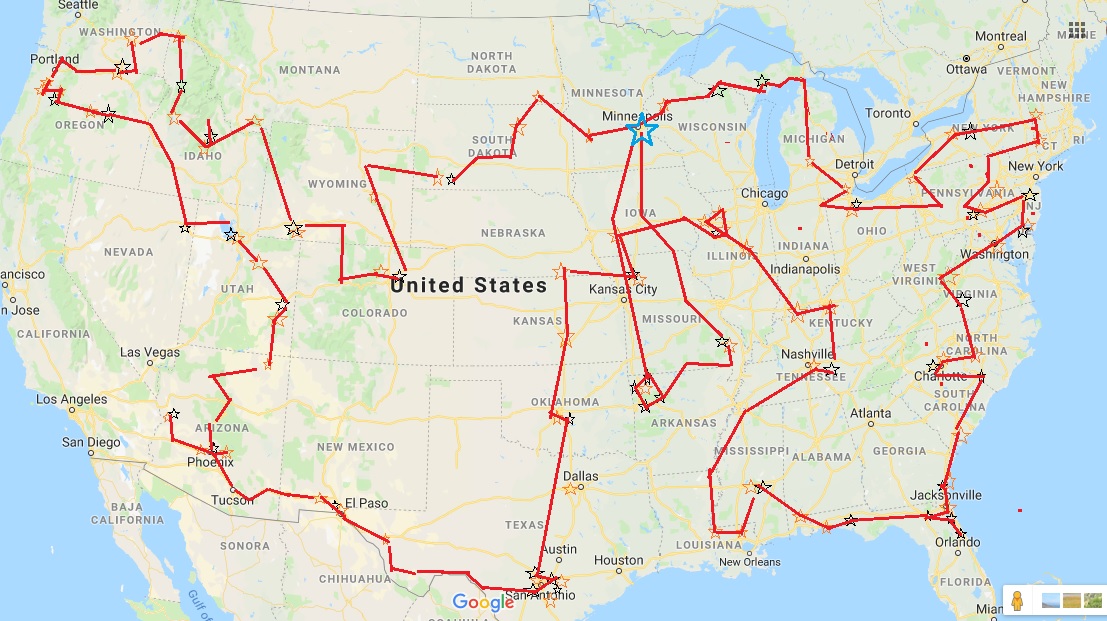A detailed satellite photo of the contiguous United States showcases a comprehensive road map with distinct features. The states appear in white, with green highlighting national parks and forests. Grey lines delineate state boundaries, while prominent yellow lines trace the interstates. The map suggests a grand road trip plan across the lower 48 states, skimming the borders of Mexico and Canada with the adjacent oceans providing a natural frame.

At the center, an aqua star marks the starting point near Minneapolis, Minnesota. From this origin, red lines chart a zigzagging journey through several states. The trip begins by heading eastward into Wisconsin, continues to the Upper Peninsula of Michigan, and moves onward through Ohio. The path then stretches northeast to New York and Pennsylvania before turning south down the East Coast, reaching as far as Jacksonville and Orlando, Florida. 

The route then reverses back north through Mississippi and Louisiana before moving up through Nashville, Tennessee, and Illinois. It dips south again into Kansas City, traversing Nebraska, Kansas, and Oklahoma. The southern leg skims past Dallas and Houston, Texas, and further down to San Antonio, then veers left to El Paso. 

The adventure continues west to Phoenix, Arizona, then northward through Utah, skirting the corners of Nevada and Idaho to Oregon and Portland. It extends further to Washington state, back through Idaho, Wyoming, Colorado, South Dakota, and the edge of North Dakota, eventually looping back to Minneapolis.

Additionally, a smaller loop is marked starting from Minneapolis, heading south through Iowa to Kansas City, Missouri, forming a circular route before returning to Minneapolis. This intricate map highlights an epic road trip, meticulously planned to cover a vast swath of the United States.